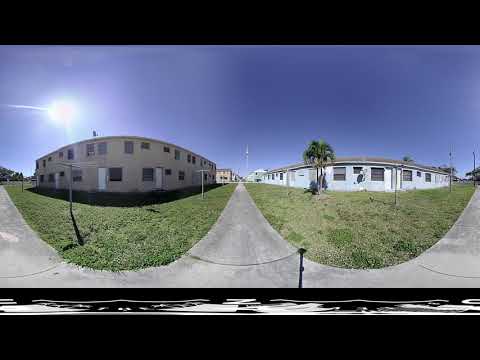The skewed photograph showcases an outdoor scene featuring two apartment buildings amidst a residential or possibly old army barracks setting. On the left, a beige, two-story building stands, while to the right, a blue, single-story building is seen with a lone palm tree in front. The image is vibrant with a bright blue sky and the Sun positioned to the left. The buildings are part of a long row, with the left side consistently two-story and the right side single-story, all painted in similar colors. Grass and walkways surround the buildings, with walkways visible on the left, right, and middle. A chain-link fence with a rope hanging marks the beginning of the walkway, and a vague telephone or clothing line crisscrosses near the buildings. The photograph lacks any text or identifying information about the location, time, or photographer. The setting is bathed in daylight, highlighting various colors such as shades of green for the grass, tan and beige for the buildings, and light blue for the clear sky.